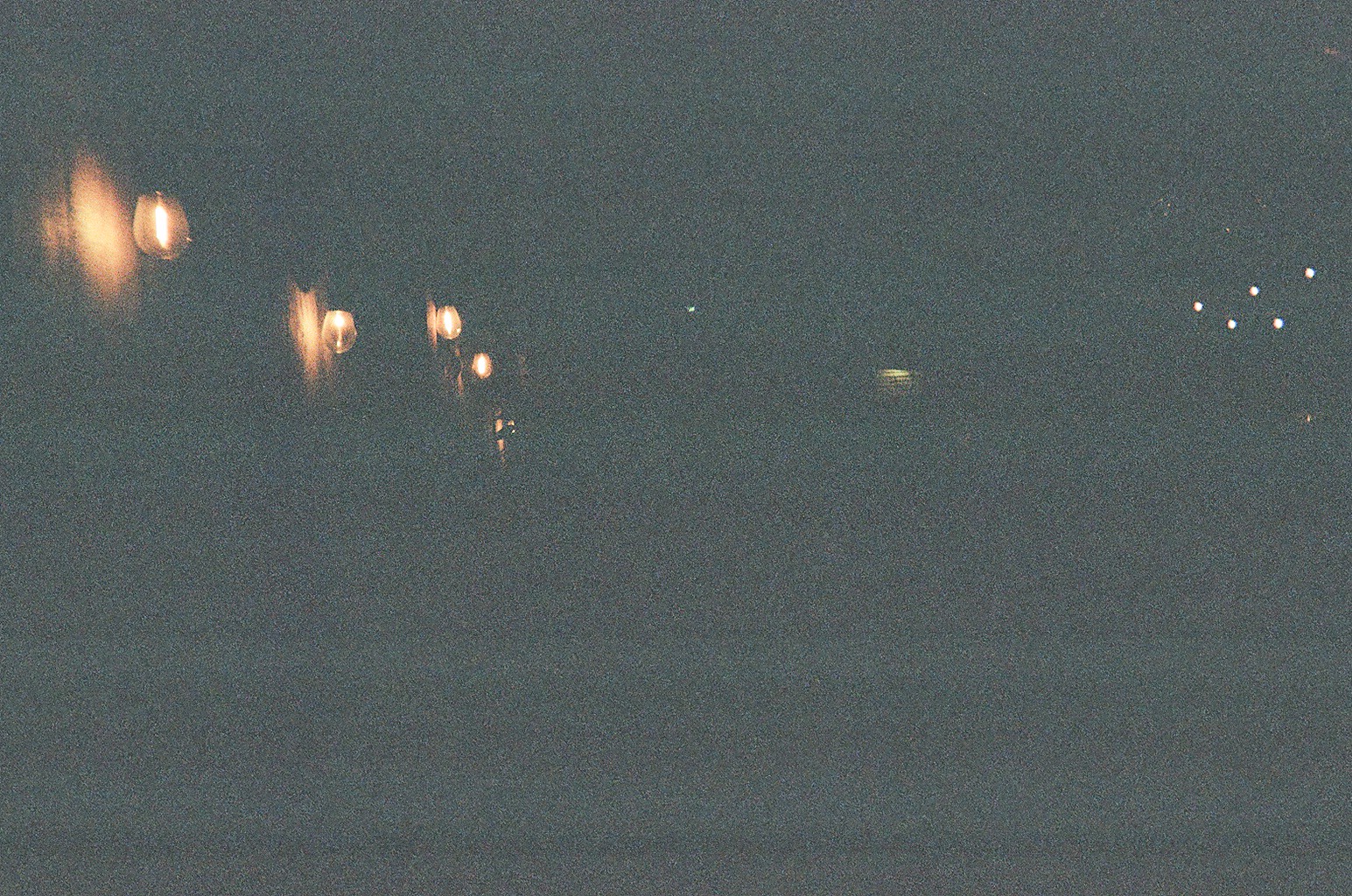In this atmospheric nighttime photograph, the low-light setting reveals a captivating array of scattered light sources against a predominantly dark and grainy background. The image, though lacking in clarity, highlights various soft, glowing spots that differ in intensity and size, hinting at potential origins like distant buildings, street lamps, or reflections on water. Towards the right side of the image, a cluster of smaller, brighter white lights captures attention, their precise nature—whether distant urban lights or stars—remaining ambiguous due to the photograph's grainy texture. Overall, the picture evokes a mysterious, almost ethereal mood, leaving much to the viewer's imagination.